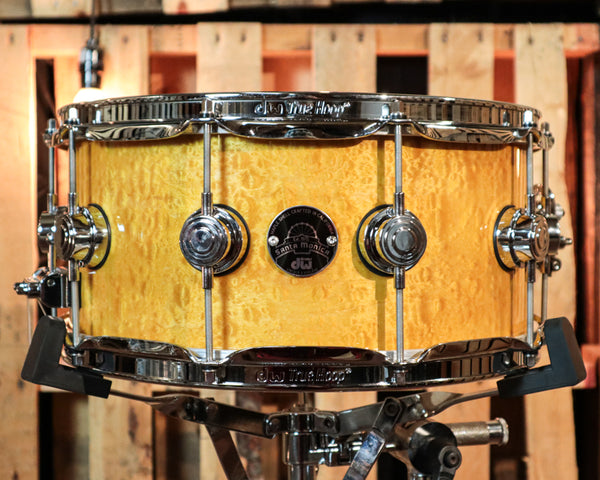A detailed side profile photograph of a snare drum placed at the center of the image, showcasing its striking design. The drum features a shiny, light wood veneer with an intricate, glossy finish that has a slightly bubbly appearance. Both the upper and lower rims of the drum are made of silver metal, complete with engraved writing. Supporting metal rods run vertically and horizontally between these rims. Centrally located on the wooden body of the drum is a circular metal logo that reads "Santa Monica" above "DW." The background consists of a wooden pallet with vertical slats and light gaps, adorned with various internal lights that create a blurred, warm ambiance. The drum is mounted on a stand with small, black L-shaped handles supporting its edge. The stand itself is crafted from silver metal. The entire composition captures the elegance and craftsmanship of the drum against a rustic wooden backdrop.